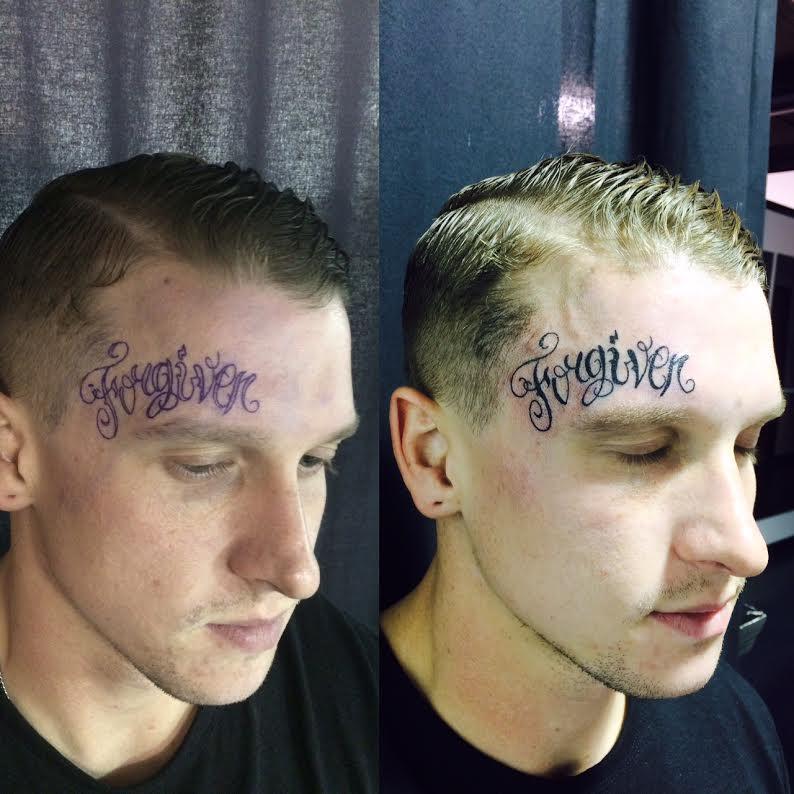This square photograph presents a "before and after" sequence of a man captured in a tattoo parlor, each image showcasing him from the neck up as he sits sideways. In the left image, behind him is a light gray curtain. He is clean-shaven, with blonde hair parted to the side, and is wearing a blue shirt. The stencil of the tattoo, "forgiven" in a scrolly script, appears in purple ink along his right forehead, from his temple just above his eyebrow, indicating the outline of the tattoo to come.

In the right image, the man is positioned against a slightly different backdrop: a blue curtain with a visible black ceiling and a black and white wall. The tattoo, now completed, is in black ink, with remnants of pink around the edges suggesting recent work and mild swelling. His eyes are closed, and he sports slightly more stubble than in the first image. He wears another blue shirt, indicating a possible time lapse between the two photos. The tattoo "forgiven," scripted gracefully along his right forehead, contrasts dramatically from its earlier stencil form.